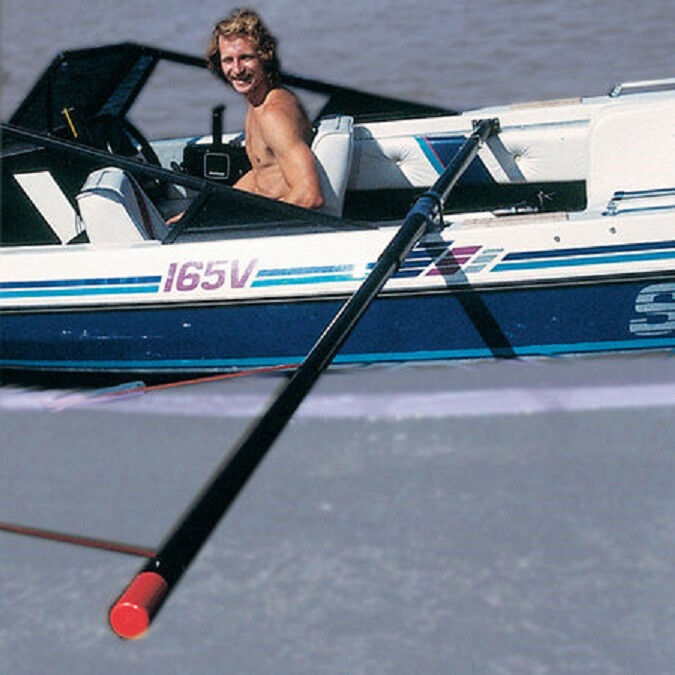The photograph depicts a shirtless man with curly blonde hair and a thick mustache sitting in the driver's seat of a small, open-top speed boat. The boat is primarily blue and white, featuring distinct markings including "165 V" and small rectangular designs in raspberry and blue. In front of the man, who is smiling and looking at the camera, is a steering wheel, indicating he is at the helm. Despite the overall low quality of the image, details such as a black metal pole with a red cap extending towards the viewer and the juxtaposition of pavement or dock in the foreground with water in the background are evident. These elements suggest the boat is moored or docked rather than in motion.